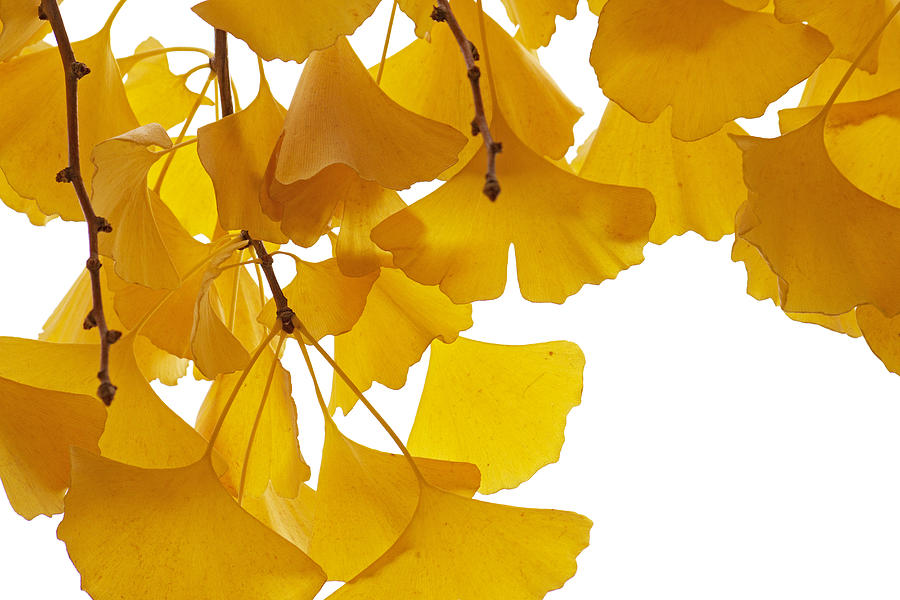This captivating nature photograph showcases an artistic display of golden yellow ginkgo leaves set against a crisp white background. The leaves, which exhibit a delicate, fan-like shape reminiscent of butterfly wings, are attached to several branch tips primarily located on the upper left side of the image. Each branch tip features clusters of three or four leaves that gently droop and point downwards. The translucent character of the leaves allows the intricate veins to be visible, with some areas appearing darker gold where the leaves overlap, casting subtle shadows. The stems, adorned with small nubs where new growth may emerge, add to the refined texture of the composition. The serene, almost ethereal quality of the image is punctuated by the occasional irregularities in the leaves, such as slight rips or missing parts, suggesting the influence of natural elements like wind or wildlife. This detailed portrayal focuses on the unique, serene beauty of ginkgo leaves, elevated by their striking color and elegant form.